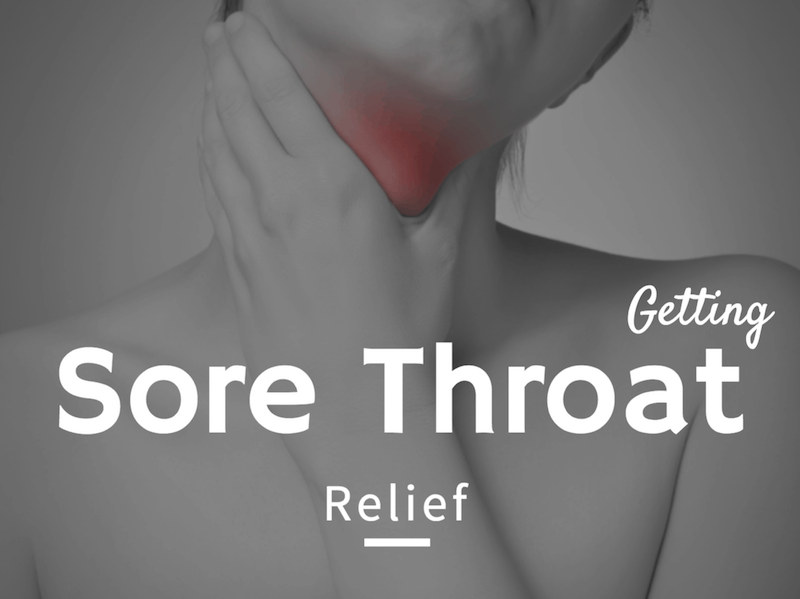The black-and-white graphic image features a partially visible woman, seemingly unclothed, against a gradient grey background. Her head tilted to one side, with her face cut off just below the mouth, reveals only her neck, part of her shoulders, and upper chest. A striking red glow highlights her throat, indicating pain. Her left hand is gently gripping her neck. Dominating the visual element, text in all-white capital letters reads "SHORT THROAT RELIEF," with "SHORT THROAT" positioned centrally near the bottom, and "RELIEF" slightly lower with a thin white line beneath it for emphasis. The word "GETTING" floats above and to the right of "SHORT THROAT," overlaying part of "THROAT." The composition suggests a medical context, possibly for a health website or advertisement focused on alleviating sore throats.